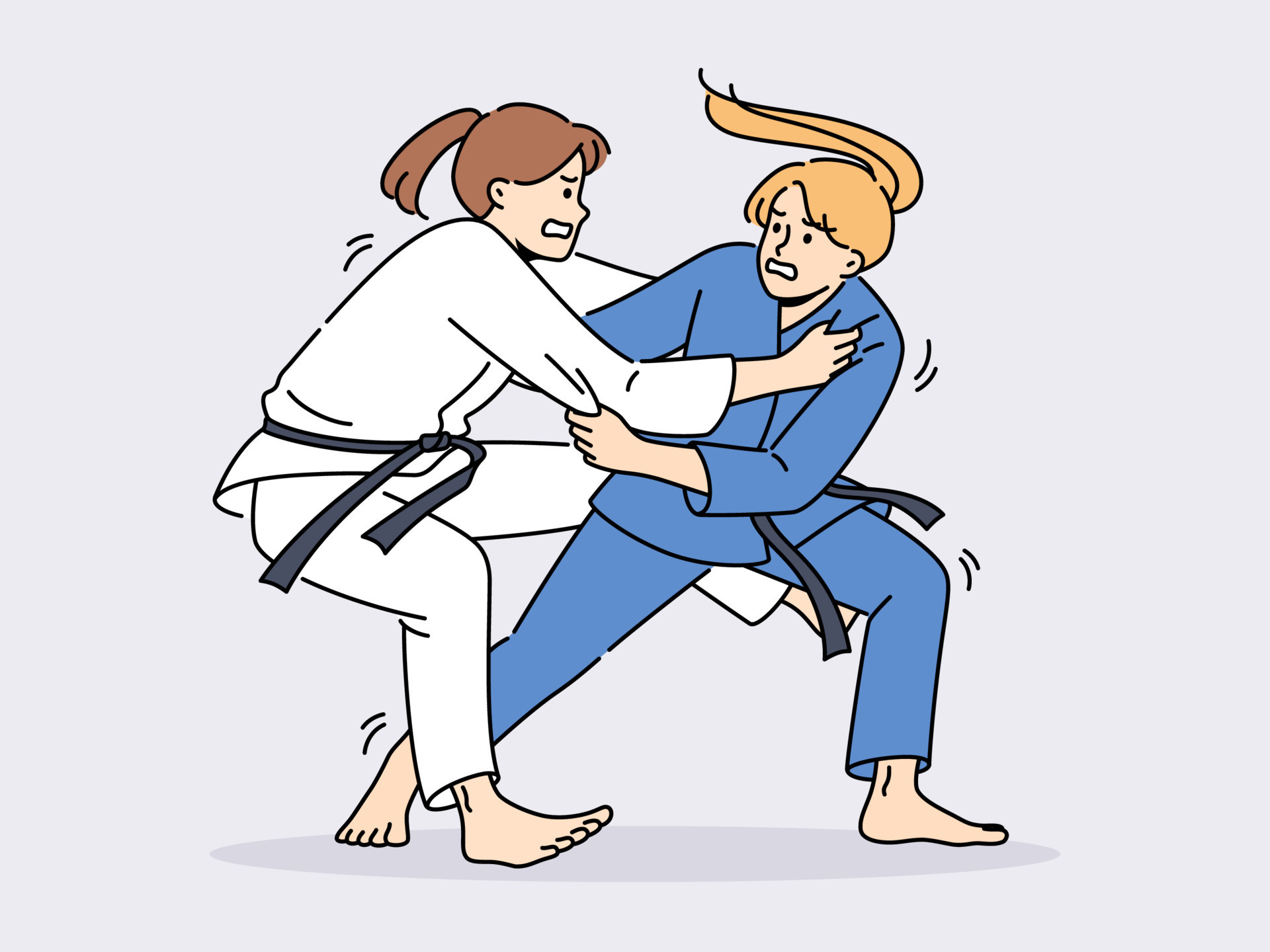This is a detailed cartoon drawing in the style of a coloring book, depicting two women engaged in a dynamic karate match. Set against a light blue backdrop, the women are positioned dead center, locked in an intense moment of action. On the left stands a woman with short brown hair, her back oriented to the left side of the image while her grimacing face is pointed to the right. She dons a traditional white gi with a blue belt and no shoes. Her right hand clutches the left shoulder of her opponent, while her left leg is raised behind the woman in blue, balancing precariously on her right leg as if she's about to be thrown.

Facing the camera is her opponent, a blonde woman with her long hair tied into a side ponytail. She wears a blue gi, also with a blue belt, and is similarly barefoot. The blonde woman's left hand grips the elbow area of the brown-haired woman's gi. Her left foot is planted firmly on the ground, toes pointing to the right for stability, while her right leg extends straight out between her opponent's legs with toes directed towards the viewer. Both women wear expressions of intense concentration, capturing the high energy and movement of their martial arts encounter.